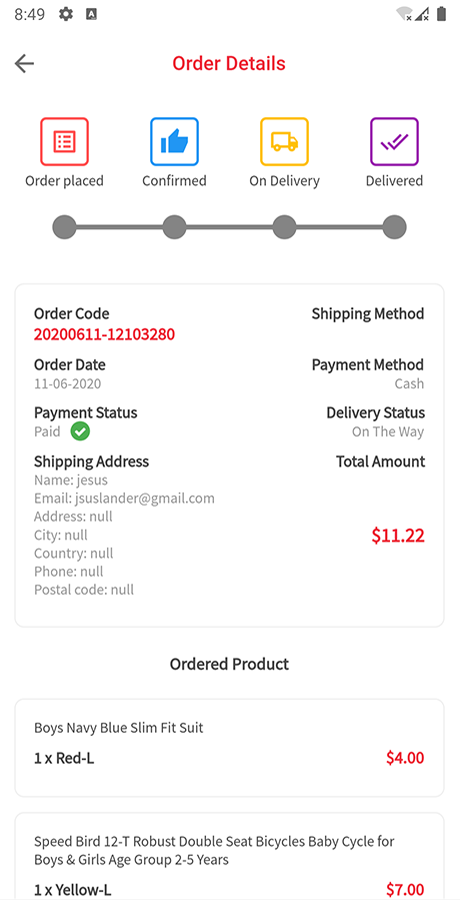Screenshot of a Smartphone App Displaying Order Details

At the top of the screenshot, the typical smartphone status bar is visible, showing the time (8:49), signal strength for Wi-Fi and network, and battery level icons. The screen is titled "Order Details" with a back arrow, indicating the option to navigate to a previous screen.

Below the title, a progress tracker with four icons - "Order Placed," "Confirmed," "On Delivery," and "Delivered" - visually represents the current status of the order, with the "On Delivery" stage highlighted.

A detailed window provides the following information:
- **Order Code:** 202611-121-03280
- **Order Date:** 11-06-2020
- **Payment Status:** Paid (indicated by a green checkmark)
  
The shipping details are somewhat incomplete:
- **Name:** Jesus
- **Email:** jsuslander@gmail.com
- **Address:** null
- **City:** null
- **Country:** null
- **Phone:** null
- **Postal Code:** null

While the "Shipping Method" field is blank, the "Payment Method" is listed as cash, and the "Delivery Status" is marked as "On the way." The total amount due for the order is $11.22.

The ordered products are listed in separate sections:
1. **Boys Navy Blue Slim Fit Suit:**
   - Quantity: 1x
   - Color: Red (confusingly labeled as navy blue)
   - Size: L
   - Price: $4.00

2. **Speedbird 12-T Robust Double Seat Bicycles:**
   - Description: Baby cycle for boys and girls, age group 2 to 5 years
   - Color: Yellow
   - Size: L
   - Quantity: 1x
   - Price: $7.00